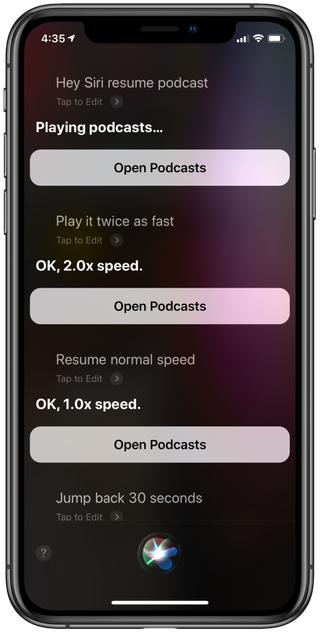The image captures an Android smartphone with a rounded design and various interface elements displayed on its screen. At the top left corner, the screen shows the time "4:35" followed by an arrow icon. On the top right, there are icons for connectivity bars, Wi-Fi signal strength, and the battery indicator.

The main part of the screen displays voice command suggestions for controlling podcast playback using Siri. These suggestions include:
- "Hey Siri, resume podcast."
- "Tap to edit."
- "Playing podcast, open podcast."
- "Play it twice as fast."
- "Okay, 2.0 times speed."
- "Open podcast, resume normal speed."
- "Okay, 1.0 speed."
- "Open podcast and jump back 30 seconds."

The color scheme for these elements is predominantly black, with rounded light gray bars for the "open podcast" suggestions. Most text appears in white, except for the text within the "open podcast" bars, which is in black. The commands "Play it twice as fast," "Okay, 2.0 times speed," and "Jump back 30 seconds" are notably in white text.

At the bottom of the screen, there is a circular home button with a bright light at its center. The overall setup and appearance are typical of a standard Android phone, with a focus on podcast control functionalities.